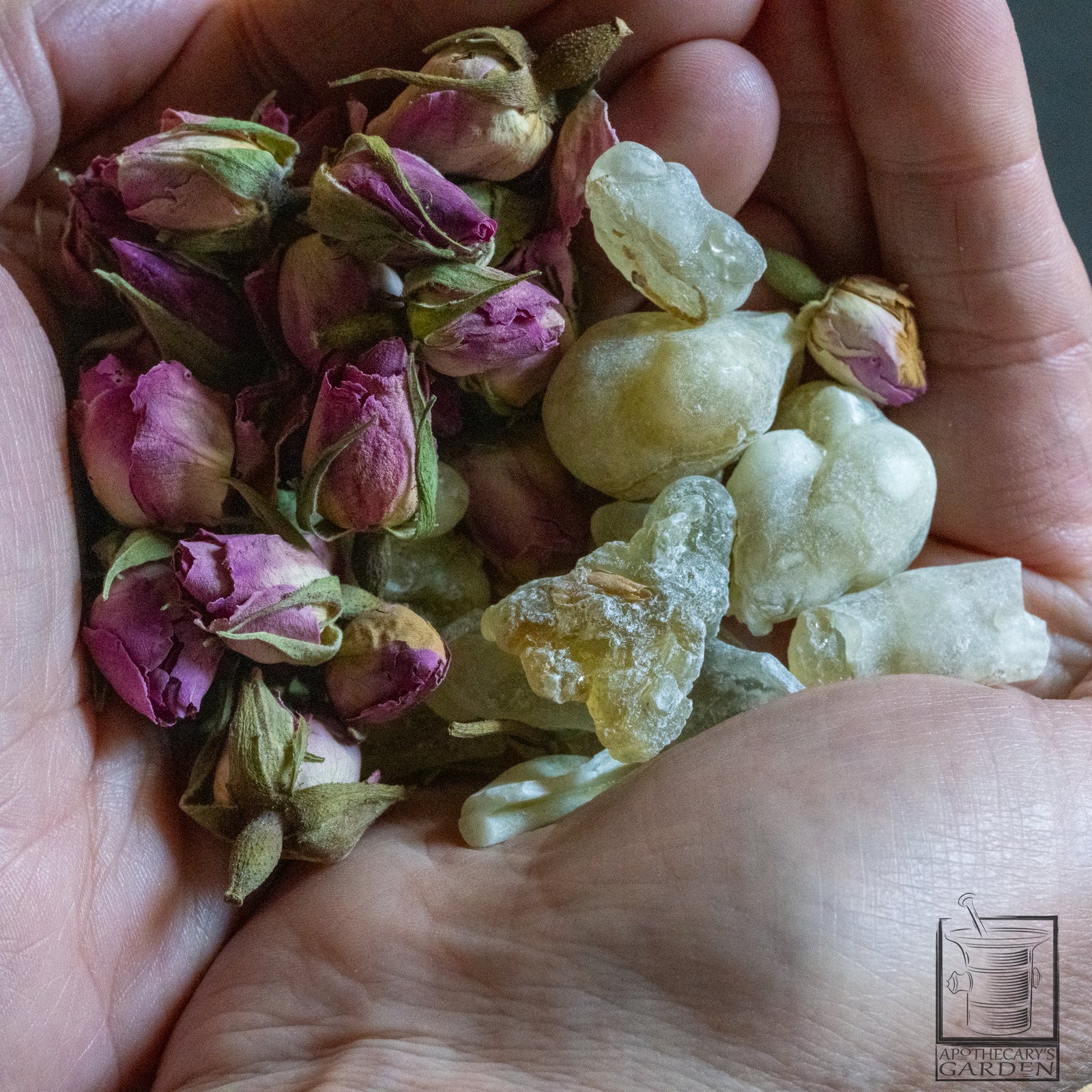This detailed indoor close-up photograph showcases a pair of cupped hands belonging to a fair-skinned person, with their left hand positioned over the right. The hands extend from the lower left corner, encompassing the entire image. Each hand holds unique items: in the left palm, there are several potpourri rosebuds, approximately a dozen, displaying a pinkish-purple hue with green stems and some dried brown leaves mixed in. Meanwhile, the right palm cradles six or seven unpolished, semi-translucent white crystals and small stones, some slightly jagged. The veins on the person’s light skin are faintly visible near the palms. In the lower right corner, an overlay logo from "Apothecary Garden" featuring a black mortar and pestle illustration adds a touch of herbal or medicinal context to the scene.